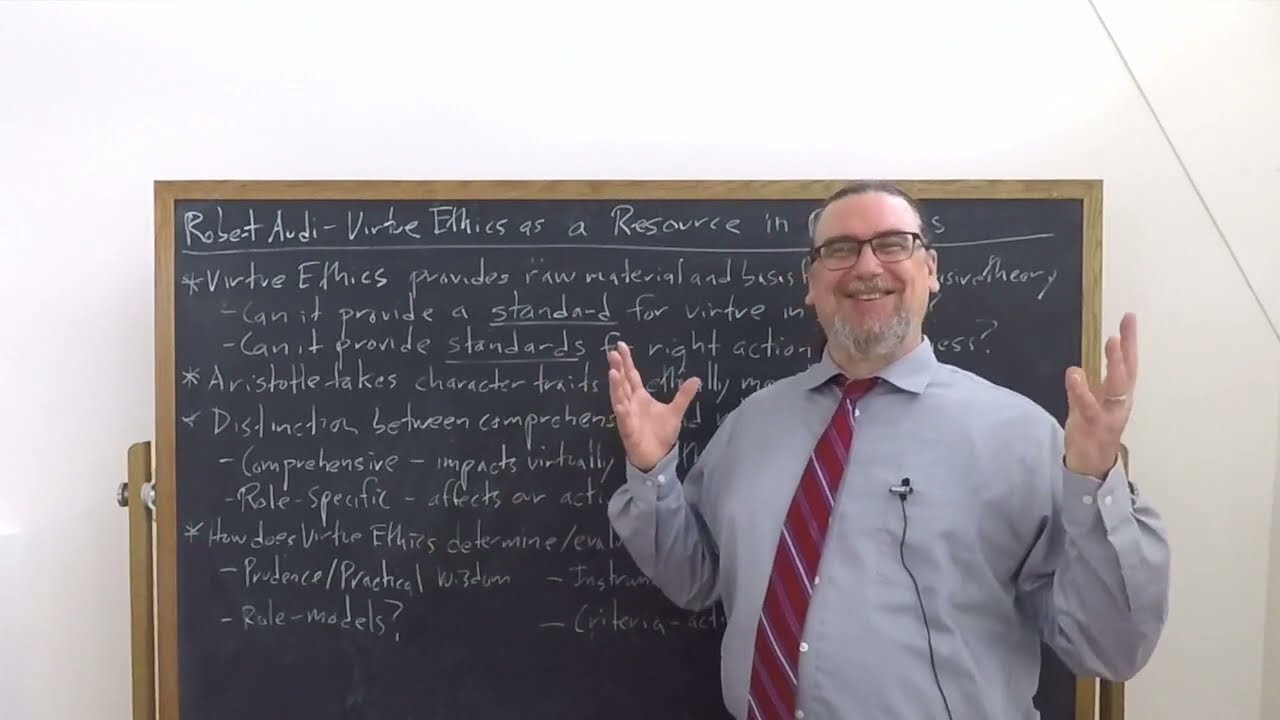The image depicts a middle-aged, heavier-set man with a gray goatee and mustache, and black-framed glasses, who appears to be instructing or leading a classroom lesson. He is wearing a long light gray button-down collared shirt paired with a red tie that features purple and white stripes. A small black lapel microphone is clipped onto the pocket of his shirt, with a wire running downwards. He is standing with both hands raised, seemingly in the middle of an explanation, and he is smiling.

This man is positioned slightly to the right of a large black chalkboard that dominates the background. The chalkboard is encased in a plain wooden frame with arms that suggest it can be flipped for dual-sided use, and it also has silver brackets visible on the sides. The chalkboard is set against an all-white wall and has numerous written notes in white chalk, many of which are obscured by the man. What's visible of the text reads “Robert Audie: Virtue Ethics as a Resource in…” followed by bullet points outlining concepts related to virtue ethics, though much of the content is partially cut off due to the man’s position. The entire scene seems to be taking place in an educational or school setting.